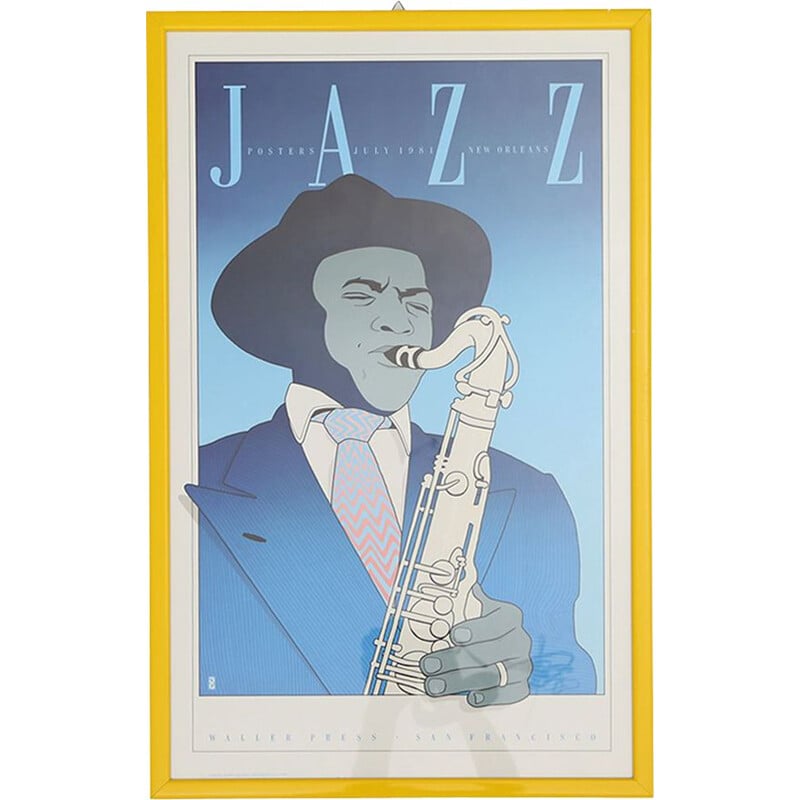The image is a sophisticated, multi-colored poster intended for wall display. It features a vertical rectangular composition with an elegant yellow frame and a gray border. The primary background is shaded in varying hues of blue, darker at the top and fading to lighter shades at the bottom. At the top center of the poster, a small hook is present, emphasizing its design as a hangable piece of art.

Prominently displayed across the top section of the darker blue area is the word "JAZZ" in large, all-uppercase light blue letters. Between these letters, the text "Fosters, July 1981, New Orleans" is interspersed. Below this, the poster depicts a meticulously detailed illustration of a black man, exuding a sense of musical passion. He is dressed in a stylish black fedora, a crisp white shirt paired with a tie, and a refined blue suit. The man is deeply engrossed in his performance, playing a saxophone with his eyes closed, and notably, he adorns a wedding ring on his finger. Beneath this vivid artwork is additional text on a white background that appears to read, "Waller Press, San Francisco," adding a final touch of refinement to the piece.